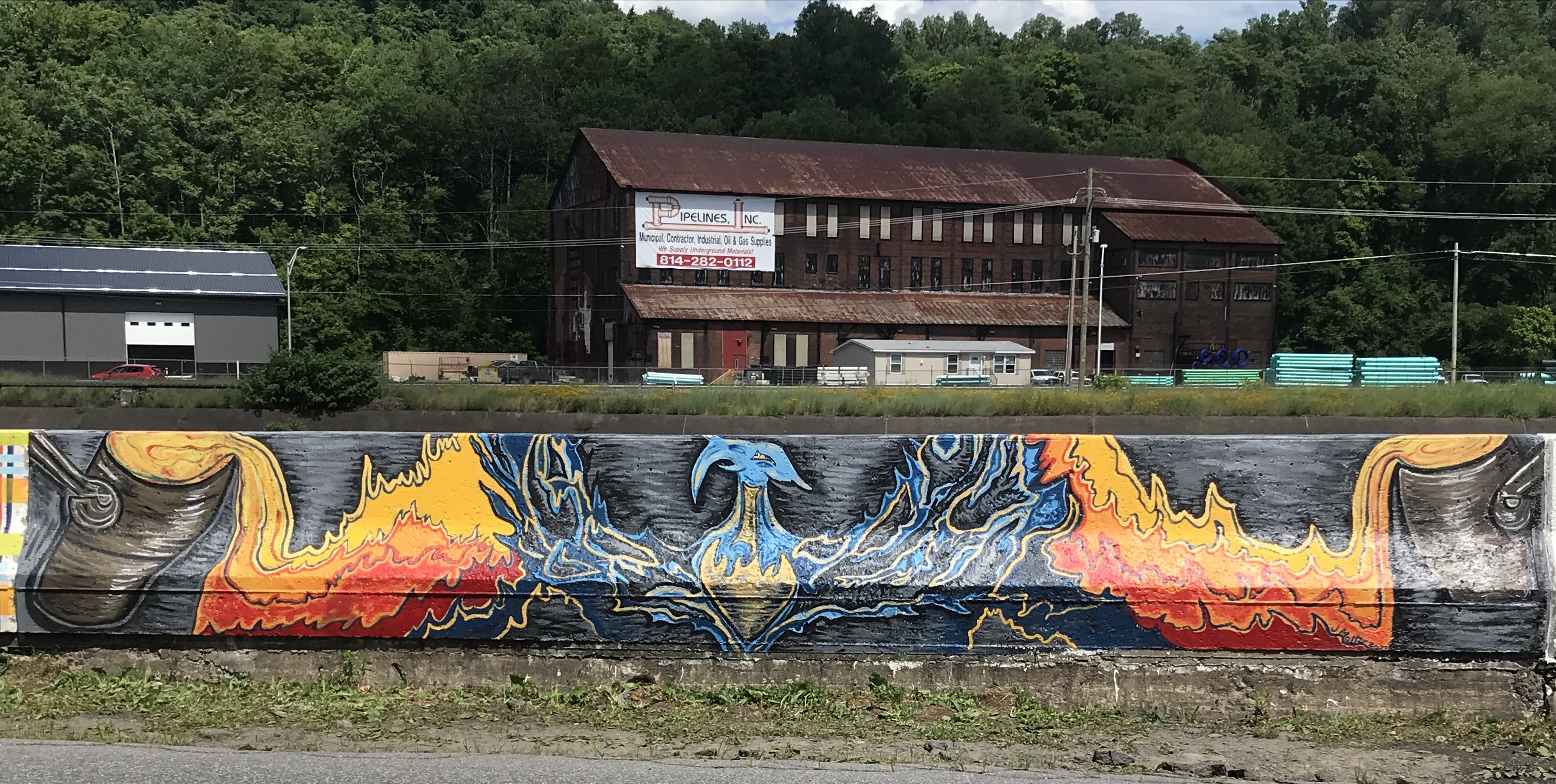The image depicts a vibrant, detailed mural adorning a long concrete barrier in an outdoor setting. The mural features dynamic, orange and gold flames emerging from gray barrels or machines, converging towards the center to form a magnificent blue, bird-like creature reminiscent of a phoenix, seemingly made of electricity. The background of the mural has a silver and gray hue that gives it a subtle, fluorescent quality. The mural is bordered by a stretch of asphalt and a small patch of grass.

In the background, several buildings can be seen, including a large, rundown old factory with faded reddish-brown walls and a rusty tin roof. This building appears to host a sign that reads "Pipelines, Inc.," though the text is somewhat unclear. Nearby, there is a smaller, gray building with a garage door partly open, in front of which a red car is parked. A tan-colored trailer-like structure and an additional factory building also feature in the scene, alongside various power lines. Thick green woods populate the distant background, adding a touch of nature to the otherwise industrial environment. On the right side of the image, some green, bus-like objects can be observed, though their exact nature is ambiguous.